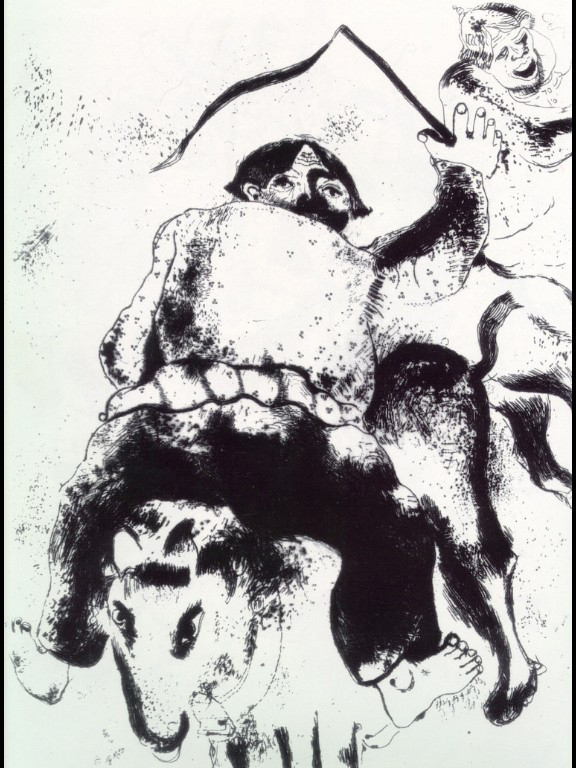The black-and-white, stylized drawing on plain white paper features a rotund man with a peculiar, oddly fat face and short hair, riding backward atop an ambiguous animal, which could be a horse, mule, or even a wolf. The man is wearing black pants, bare feet, and a robust shirt, and has one hand holding a whip. Positioned behind him, at the upper right corner of the image, is a disturbing, monkey-like creature with an open mouth, appearing to laugh at the scene. The man's backward orientation and the undefined nature of the animal add to the surreal and odd nature of the composition.